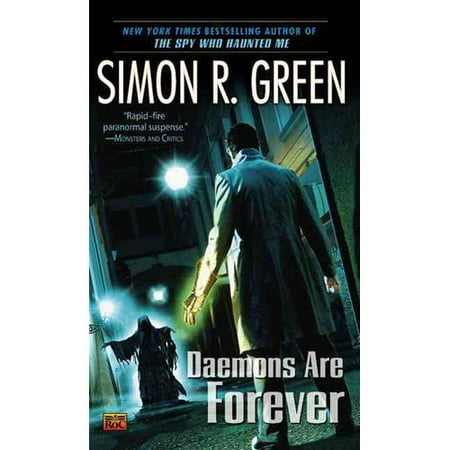The book cover, in a dark, noir alleyway with hints of blues and greens, features a haunting scene where a man in a beige trench coat, standing with arms outstretched, faces a ghoulish figure at the end of the street. Illuminated by a glowing white and blue light, the eerie figure casts a shadow. The title, "Demons Are Forever," is positioned at the bottom right in white font, with the author's name, Simon R. Green, displayed prominently above in large white letters. At the top, the text reads, "New York Times Bestselling Author of The Spy Who Haunted Me," in a gradient from light blue to darker blue. The cover also includes a review stating "Rapid Fire Paranormal Suspense" and a mention of "Monsters and Critics." The entire layout, from the text positions to the spooky imagery, evokes a chilling horror setting that perfectly encapsulates the paranormal suspense genre.